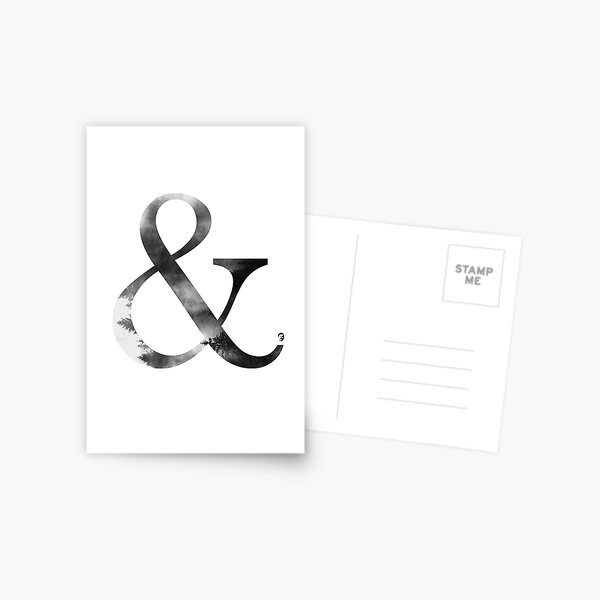This image features the front and back of a white postcard against a very light gray, almost off-white, background. Centered on the left side is a vertical rectangle showing the front of the postcard. Dominating the center of this side is a large, artistically faded gray-and-black ampersand symbol (&), resembling an 'S' shape with subtle leaf patterns at its curves. Adjacent to the left, and slightly overlapping the right portion of the postcard's front, is the back side of the postcard positioned horizontally. The back side displays a square in the upper right corner with the text "Stamp Me" centered inside it, rendered in a slightly darker gray. Below this square are four evenly spaced, light gray horizontal lines, presumably for writing an address or message. A vertical line divides the left and right sections of this side, but it is partially obscured by the overlapping front of the postcard. The image collectively highlights the interplay between the front and back designs of the postcard, with careful attention to the distinct graphical elements and subtle shades of gray.